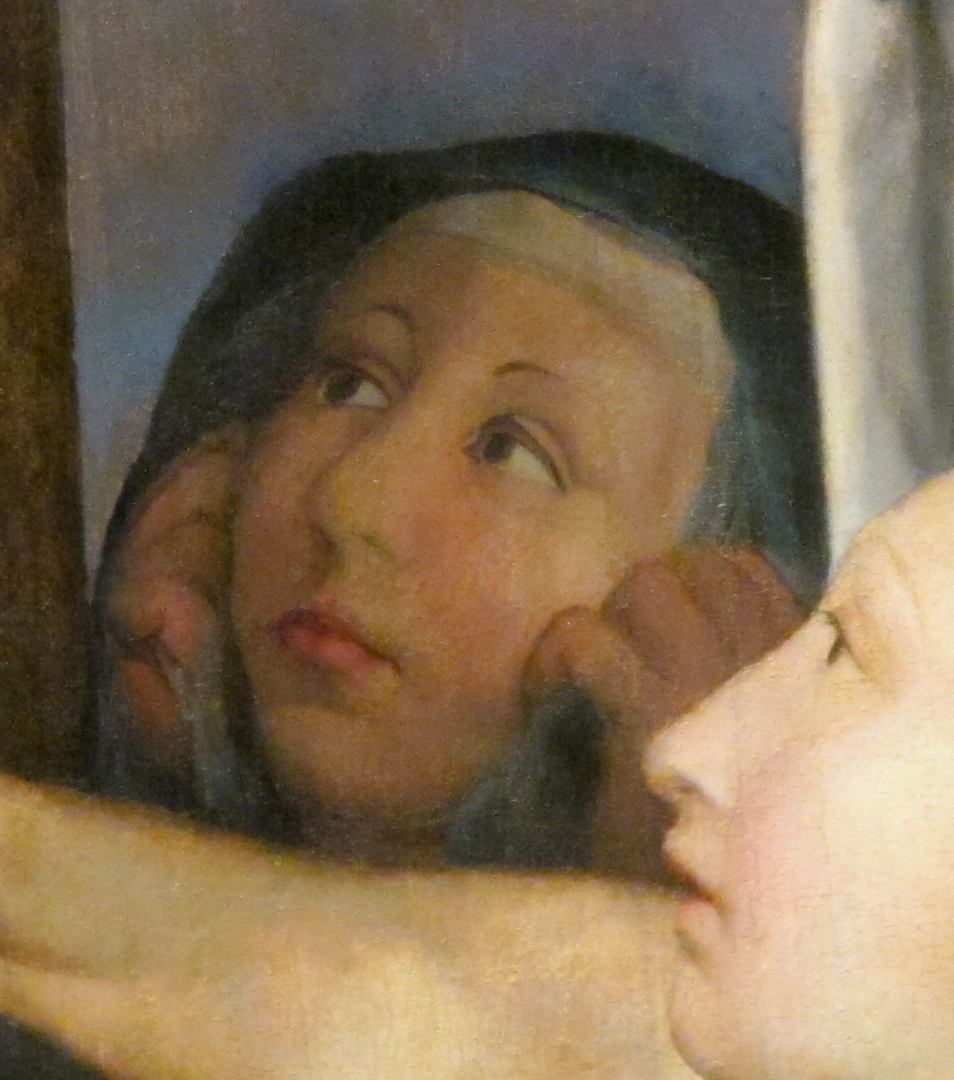The artwork showcases two women rendered with exquisite detail, potentially reminiscent of Renaissance painting techniques. In the bottom right corner of the composition, there is a profile view of a woman with very fair skin, slightly reddish cheeks, and brown eyes. Her arm stretches forward towards the left, and although her hairline is not visible, her placement within the painting suggests a somewhat contemplative mood. Behind and slightly above her, another woman is depicted, also with very fair skin, pink lips, and striking blue eyes. She wears a blue headdress, with a white strip visible at her hairline. Her hands, which appear to have a purplish hue, clutch the headdress, and her fingers press gently against her cheeks as she gazes contemplatively upward to the left. The background of the image transitions from blue to white as it ascends, with a white curtain hanging down behind the woman in the background. The overall composition, characterized by soft lines and subtle shading, creates an impression of longing or introspection, capturing a moment frozen in time with a classical, timeless quality.